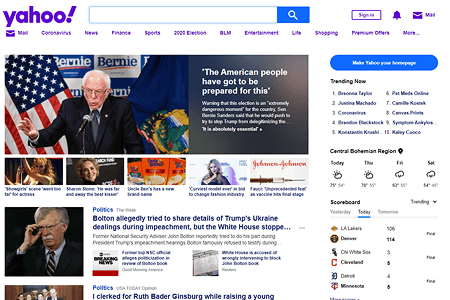The Yahoo homepage is prominently displayed, showcasing the classic minimalist design of the platform. 

In the top left corner, the iconic Yahoo logo in purple draws immediate attention. Centered below the logo is an empty search bar accompanied by a blue button adorned with a magnifying glass icon, inviting users to begin their search. Adjacent to the search bar, a series of essential icons are strategically placed: a 'Sign In' button, a bell icon for notifications, and a mail icon, ensuring quick access to vital features. 

Just beneath this row, a horizontal navigation bar presents various tabs, guiding users to different sections such as Mail, News, Finance, Sports, BLM, Entertainment, and Life.

Dominating the main section of the page is a notable image featuring Bernie Sanders. To the right of Sanders' picture, a caption reads, "The American people have got to be prepared for this," accompanied by a brief paragraph of white text, providing context to the image.

Further down, a series of eye-catching thumbnails are aligned, each with enticing visuals and descriptive text, offering a snapshot of various trending stories. The bottom left corner features a larger image with a partial headline about John Bolton: "Bolton allegedly tried to share details of Trump's Ukraine dealings during impeachment, but the White House stopped," indicating a significant news piece but with the headline truncated.

To the right, a prominent blue button encourages users to "Make Yahoo your homepage," fostering a deeper connection to the site. Below this call-to-action, trending topics are highlighted, including "Central Bohemian Region" and a "Scoreboard," catering to users' diverse interests.

The layout and elements together create a comprehensive, user-friendly homepage, effectively integrating news, personal utilities, and navigation.